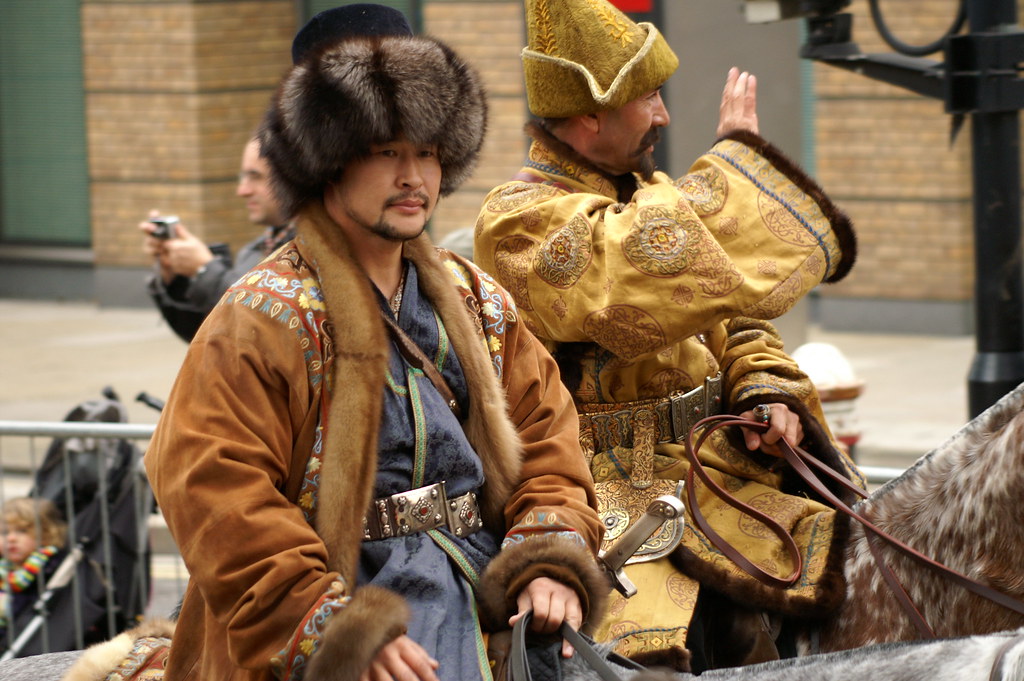This vibrant photo depicts a lively parade scene with two strikingly dressed men riding their respective horses at the forefront. The central focus is on the man closest to the camera, who exhibits an Oriental heritage and sports a prominent mustache and beard. He is adorned in a rich brown, embroidered coat with intricate designs around the shoulders and cuffs, which are lined with fur. The man's hands, especially his left hand, clutch the reins of a horse that is only partially visible beneath him. His head is crowned with an impressive black and white fur cap, reminiscent of an Eskimo hat. He also wears a distinctive blue shirt with an ornate silver belt featuring a prominent buckle, and a sword handle peeking from his side adds to his grand demeanor.

Next to him, facing the same direction, is another man elegantly dressed in a golden ceremonial coat with fur lining, and a similarly adorned hat. This man, also sporting a mustache and beard, waves his right hand energetically at onlookers off camera, indicating active engagement with the parade crowd. His horse, seen with distinctive white and brown coloring, adds to the dynamic tableau. 

Behind this engaging pair, a white man with glasses is seen capturing the moment with a small camera while standing next to a stroller containing a baby. They are separated from the parade route by a steel divider. The background reveals a sidewalk and a brick building, completing the vivid snapshot of this lively and colorful parade scene.